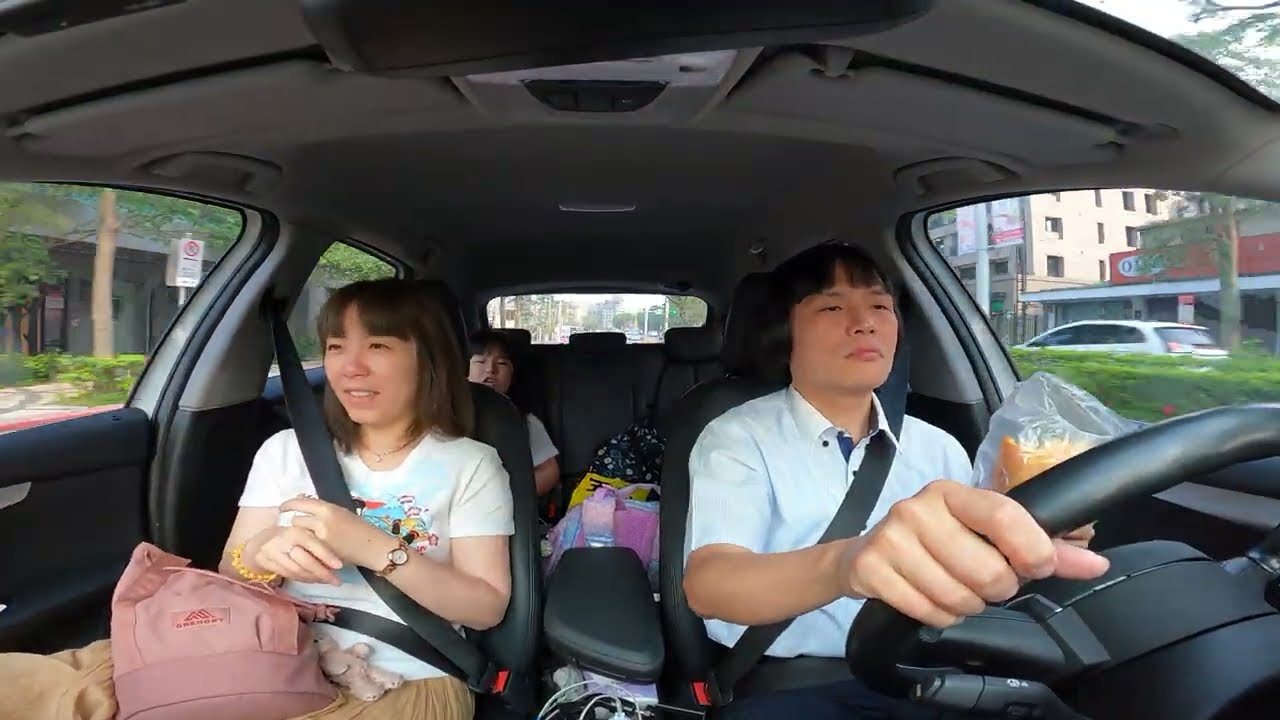The image displays a young Asian family on a drive through an urban area. The father, with medium-length hair, is at the wheel, eating a sandwich with one hand and steering with the other, dressed in a white short-sleeved shirt. He appears focused on the road, secured with a seatbelt. Beside him in the passenger seat is the mother, a young woman around 30, smiling with shoulder-length hair. She is dressed in a tan-colored dress and a white t-shirt, accessorized with a watch and a pink purse on her lap, along with a small teddy bear. From the backseat, a child, suggested to be a young boy, is visible, surrounded by several shopping bags and backpacks. The car's interior is predominantly gray and black. Through the windows, the scenery reveals bustling city streets with passing cars, buildings, businesses, bushes, and trees, indicating a typical drive through an urban or small town setting. All family members are wearing their seatbelts, and the focus of the image remains on the intimate, everyday family moment within the car.